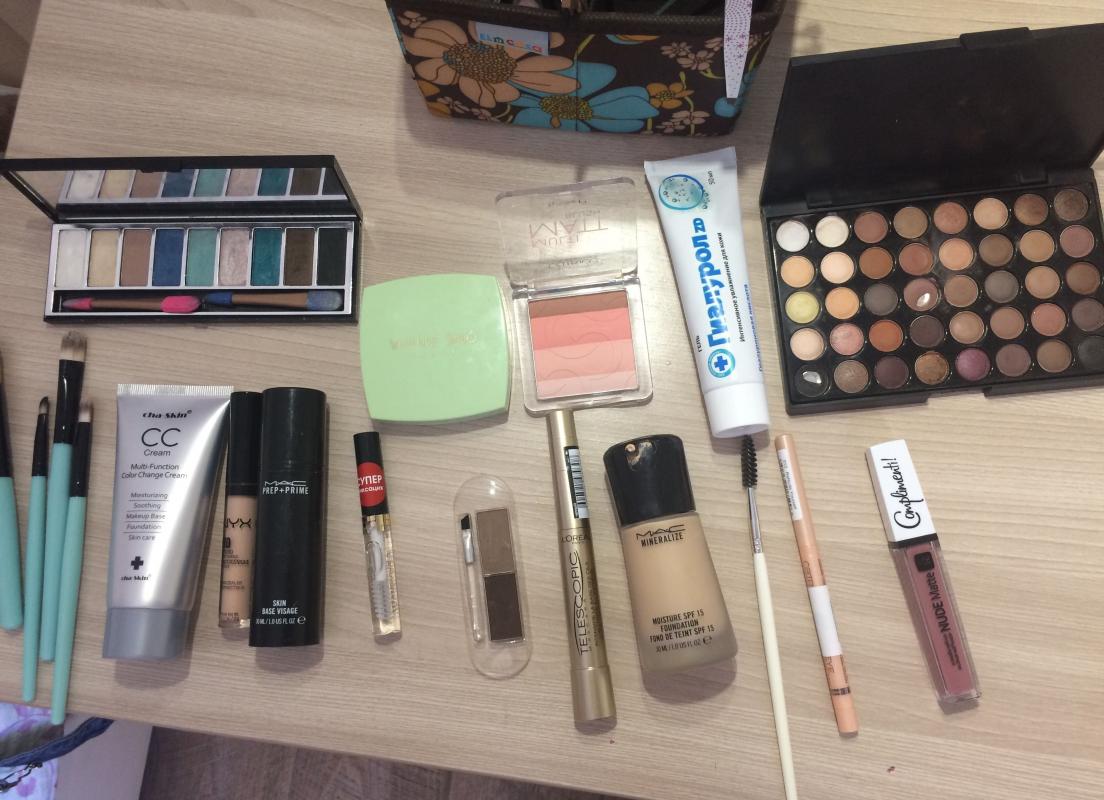The image depicts a light-colored wooden table surface, meticulously arranged with a diverse array of makeup items. On the far left, four makeup brushes of varying sizes with distinctive green and black handles are neatly laid out. Adjacent to the brushes is a sleek, silver-hued squeeze tube of cream, completed with a grey cap. Progressing rightward, there is a bottle of light brown foundation, boasting a smooth, creamy appearance. Its neighboring item is a black cylindrical bottle of primer, an essential step before applying foundation, designed to prep the skin.

Further along, the table is adorned with a mascara brush, identifiable by its sleek, elongated design. Adding a splash of color, there are several blushes that promise to bring a rosy glow, along with an assortment of eye shadows in captivating bronze and brown hues, perfect for creating versatile eye makeup looks. The collection is rounded off with a selection of lipsticks in varying shades, ready to add the finishing touch to any makeup ensemble.